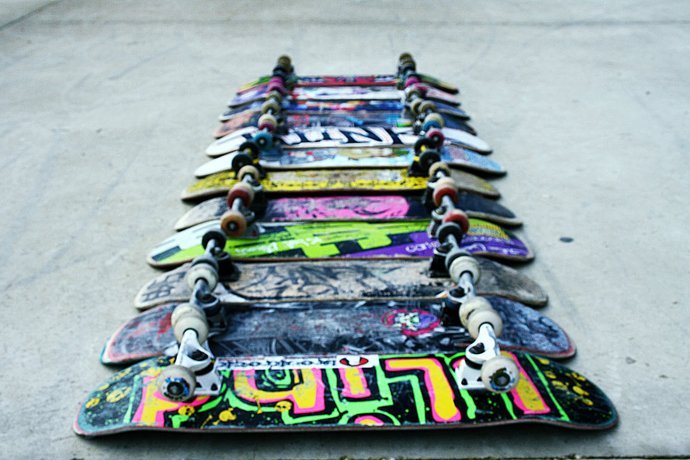This photograph showcases a lineup of 12 well-used skateboards laid upside down on a white concrete floor, revealing their wheels and trucks. Each skateboard flaunts vibrant graffiti art and varied color schemes, though the paint is chipped and the wheels are dirty, indicating they have been actively ridden. Starting from the bottom, the skateboards display a mix of colors: 
1. The bottom board features black with yellow, pink, green, and orange outlines.
2. The next one is dirty gray with a hint of red and blue in the middle.
3. The third skateboard has a grayish background adorned with graffiti.
4. Above that, a board sports lime green and purple hues.
5. The fifth board in the lineup is black with pink accents.
6. The sixth features a blackish and yellow background.
7. Next is a board with a white base accented with blue.
8. The eighth skateboard has a white background with black letters.
9. The ninth is a collage of red, blue, and black.
10. The tenth board has a mixture of yellow, red, blue, and black.
11. The eleventh board carries a white and red design.
12. Finally, the top board is a blend of red and blue with a bit of black.

These skateboards, all distinct in their graffiti designs and clearly showing signs of wear, are captured in a moment of rest before their next ride.